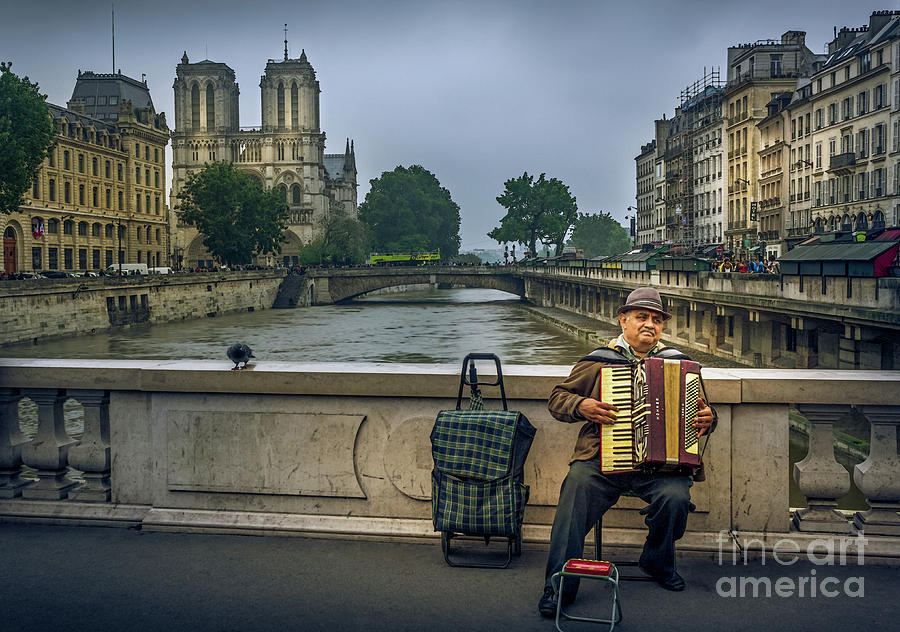This photograph by Fine Arts America showcases an old man wearing a light brown hat and a brown jacket, playing an accordion on a city street. He appears to be busking, seated on a stool with a green plaid carrying case nearby. The scene is set in a European city, possibly Amsterdam or Venice, characterized by its iconic canal running through the middle. Flanked by elegant, old European buildings with intricate architecture, including arches, filigree, and unique window shapes, the setting is both picturesque and historic. A concrete bridge spans the canal, connecting both sides of the city, with stately buildings on either side, including what looks like a beautiful old church. The sky above is gray and murky, adding a somber yet classic atmosphere to the scene. A bird is also visible to the man's left, enhancing the idyllic urban landscape.